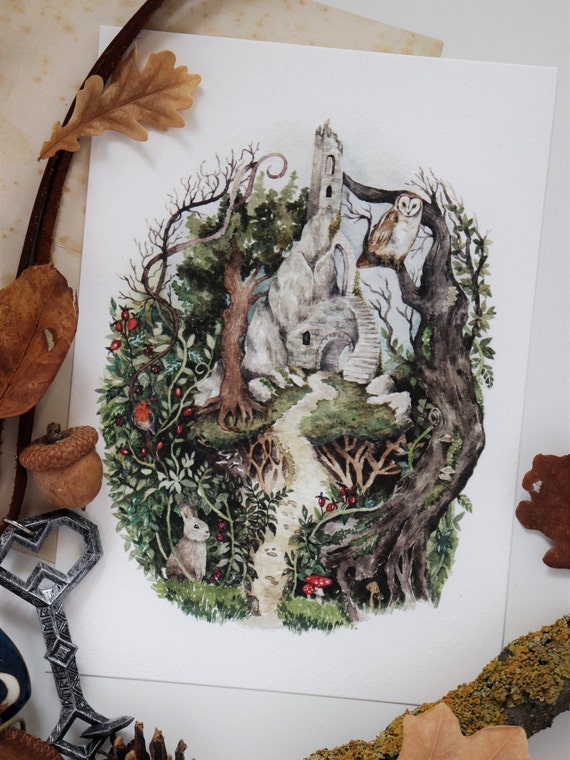The image is a detailed and fantastical drawing on a white piece of paper that lies in the center of a table. Surrounding the paper, from the bottom left and moving counterclockwise, are a variety of items: several brown leaves, an acorn, pieces of wood, and what appears to be an old-fashioned cast iron key, although its full shape isn't visible. More leaves and twigs encircle the edges of the paper. The drawing itself depicts an enchanted forest scene. On the left side, there is a lush area with abundant shrubbery, trees, a bunny, and a red bird, possibly a sparrow. Near the bottom, there are many twisted and dead vines, along with clusters of small red mushrooms. To the right, another large tree stretches upward with a brown barn owl perched at the top. In the center of the forest scene, a partially-ruined castle tower stands with a path leading towards it, surrounded by overgrowth and framed by more trees and vines. The intricate details include additional bunnies, birds, and flowers intertwined in the foliage, creating a whimsical and layered composition.